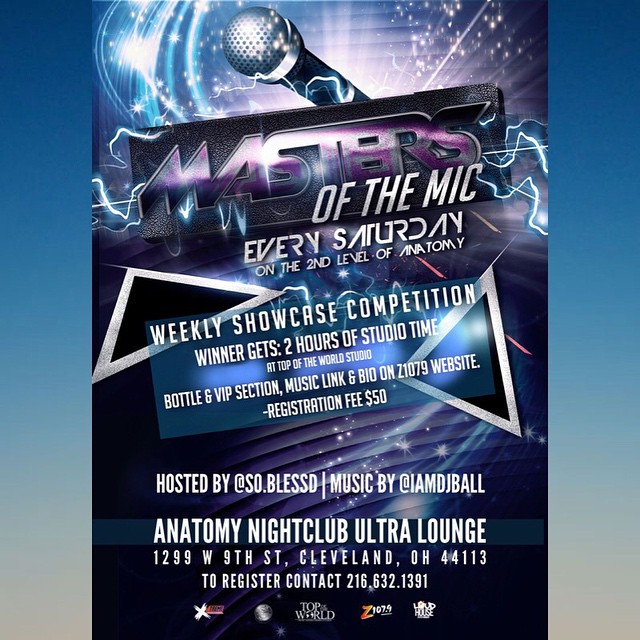The event poster prominently features a dark blue background that gradually lightens to a tan at the bottom. Overlaying this is a dynamic mix of swirling white lines, stars, light purple lightning-like stripes, and various electrical effects, creating a striking visual of energy and excitement. Central to the design is a silver microphone with a black handle. Below the microphone is a black, leather-textured rectangle with the word “Masters” in large purple letters. In smaller silver text beneath it reads, “Of The Mic,” followed by “every Saturday on the second level of Anatomy.” A light blue box underneath states in white letters, “Weekly Showcase Competition,” detailing that winners receive two hours of studio time at Top of the World Studio, bottle service in the VIP section, and a music link and bio on the Z107.9 website. It also mentions a registration fee of $50. The event takes place at the Anatomy Nightclub Ultra Lounge located at 1299 W 9th Street, Cleveland, Ohio, 44113. Additional text notes that the event is hosted by @SoBlessed with music by @IMDJBall. At the bottom of the poster are several small logos of the involved companies. Contact details for registration include the phone number 216-632-1391.